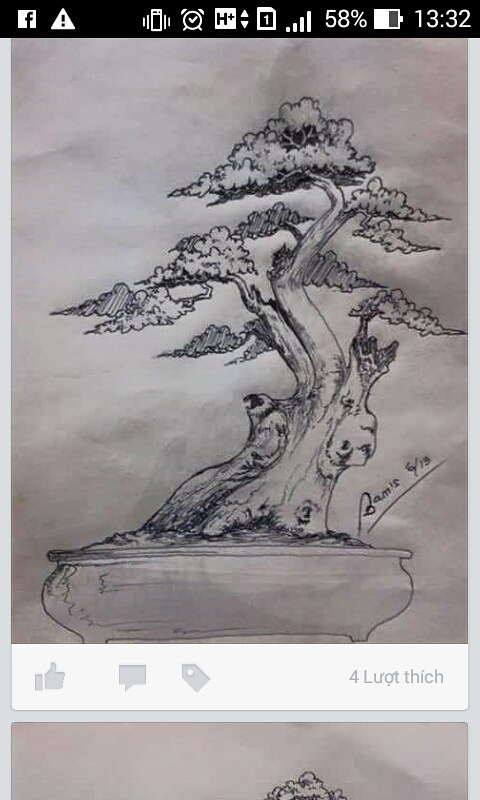This screenshot appears to be taken from a mobile phone. At the top of the screen, there is a black notification bar featuring various white icons, including a Facebook icon on the left and a small triangle with an exclamation mark. Also present are typical phone status indicators such as battery usage on the right and the time, noted at 13:32. 

The main content showcases a pencil-drawn black-and-white illustration of a tree. Directly beneath the drawing, on the right side, there's a small white bar displaying interactive gray buttons, including a thumbs-up icon along with several other symbols. Below this bar, there is text that seems to include the word "Rhinoceros", followed by the partially visible string "l-u-r-o-t" and "t-h-i-c-h".

The background features a white-to-gray gradient, resembling textured paper, enhancing the hand-drawn aesthetic of the displayed sketches and text.